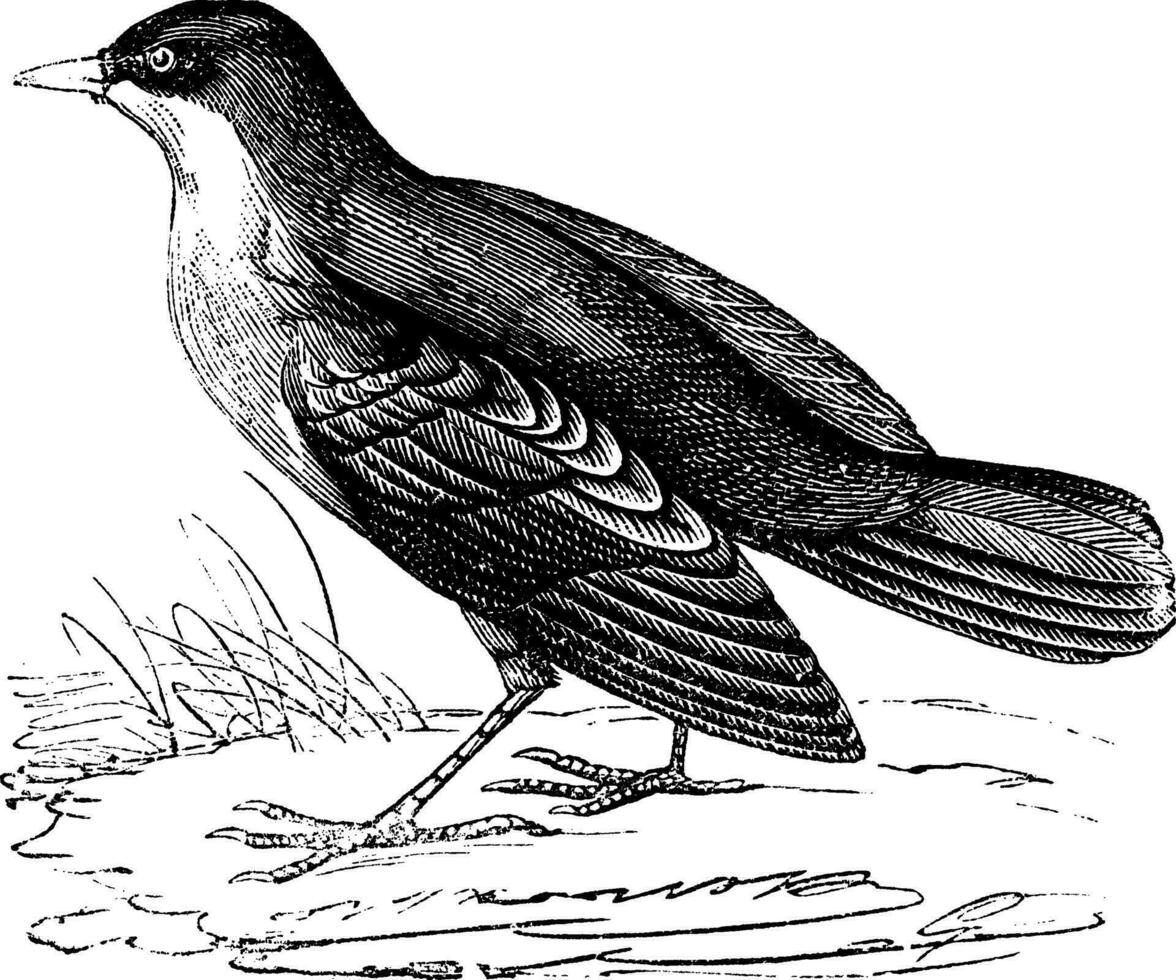The image is a detailed black and white ink drawing of a bird. The bird is oriented to the left with its head turned in that direction and its short tail feathers facing the right side of the image. It is depicted standing on a flat, squiggly-marked ground which includes indications of vegetation or grass on the left. The bird balances on two legs, each with three front toes and one back toe, all equipped with claws. The bird features a pointed beak, and its plumage on the back exhibits a lion-like pattern, contrasting with its lighter-colored stomach. The bird's wings are slightly spaced out, and there is a noticeable gap between the left wing and the tail feathers, giving the bird a unique and interesting appearance.